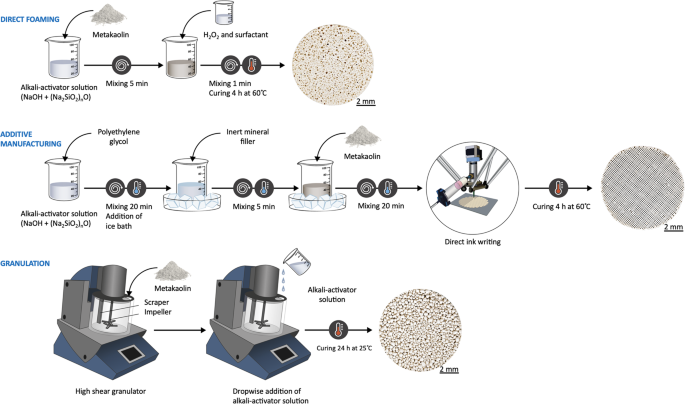The image is a detailed diagram outlining various processes related to material processing, featuring multiple illustrations and descriptive text. At the top, in blue text, it reads "Direct Foaming," accompanied by three linked illustrations. The first illustration shows a container holding a metakolin powder in an alkali activator solution. An arrow labeled "Mixing 5 minutes" leads to the next container with the mixed solution. Another arrow directs to a close-up, microscopic view of the cured solution, achieved by curing it for 4 hours at 60 degrees Celsius.

Below this section, labeled "Additive Manufacturing," the diagram elaborates further with additional containers and microscopic views. After curing, polylithene glycol is added, mixed for 20 minutes with ice bath addition, leading to further processing steps like direct ink writing. Each step is detailed with arrows and textual instructions to prepare the material for manufacturing.

The final section, labeled "Granulation," features illustrations of two blue and silver machines, described as granulators. These machines, shown with arrows, point to a microscopic view of the processed material, emphasizing a different method of breaking down the material depending on desired textures or physical properties. The entire image is a comprehensive guide to the procedures involved in producing an alkali activator solution and processing it through various manufacturing techniques.